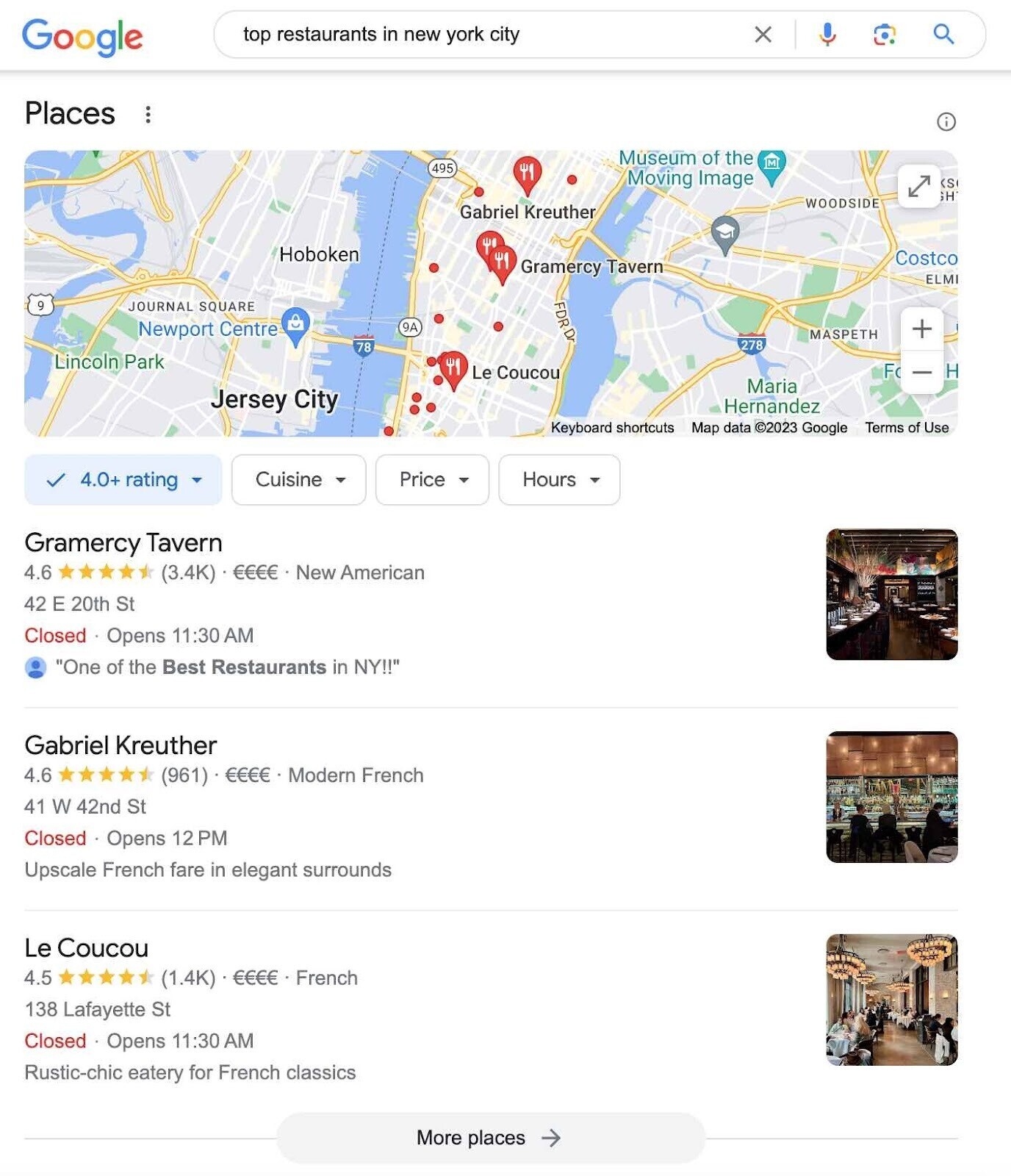The image is a screenshot from Google, featuring a search page with a clean, white background. At the top, the recognizable Google logo is displayed prominently; it consists of a capital 'G' in blue, followed by a red 'O', a gold 'O', a lowercase 'g' in blue, a green 'l', and a red 'e'. Next to the logo is an oval search bar with a dark gray border, containing the black text, "top restaurants in New York City." On the right-hand side of the search bar, there is a gray 'X' followed by a gray vertical line. Further to the right is a voice search icon, depicted as a blue pill-like shape situated within an overturned 'C' in yellow and red, with part of the base in blue or green. Additionally, there is an icon resembling a camera, divided into four colored sections—blue, yellow, red, and green—with a central blue circle. Finally, a cyan blue magnifying glass represents the search functionality.

Centered in the screen is a detailed map showcasing New York City with characteristic gray and green areas representing various buildings, and tan sections denoting different buildings and other areas. Red pins with white fork-and-knife icons signify the locations of top restaurants. A unique dark blue pin with a white shopping bag featuring a blue smiley face represents a shopping place in Jersey City, marked in bold black. A school is identified with a dark gray pin and a white graduation cap icon located on the right side. The Museum of the Moving Image is marked with a teal pin containing white details.

Highways on the map are marked with dark blue shield-like shapes highlighted with red tops: one marked '78' and another '278'. These highways connect to yellow-and-gold colored roads. The top right section of the map includes a dark gray square with directional arrows pointing left and right, as well as a rectangular section with a thin gray line separating the '+' and '-' zoom icons. 

Beneath the map, there are numerous reviews from various restaurants, providing users with additional information about dining options in New York City.